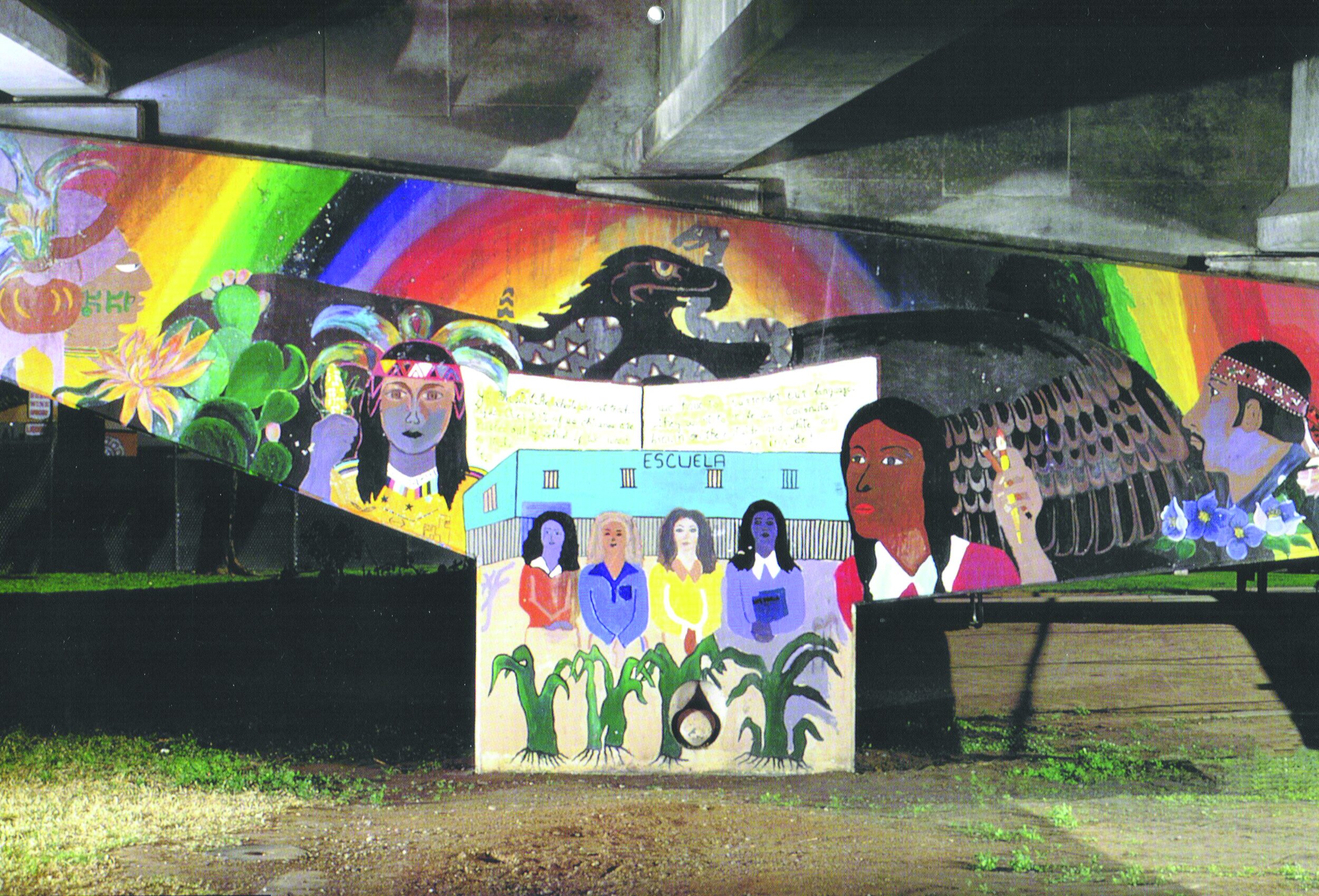This image features a vivid mural painted on concrete support beams, located underneath what appears to be a bridge or overpass. The mural showcases several interconnected scenes against a concrete backdrop, with a grassy and dirt area visible beneath it. Dominating the mural is a vividly colored rainbow with an imposing black eagle grasping a gray, white-spotted snake in its beak, its wings spread wide across the artwork. 

In the center, a square panel depicts a blue building labeled "Escuela," which means school in Spanish. In front of the building stand four figures, two of which are a bluish-purple, one white, and one light brown, with one person holding books. Four large green plants grow in front of them. To the right, a Native American-inspired purple woman with black hair wears a headdress and holds a piece of corn. On the left of the eagle, a dark-skinned girl with black hair holds two pencils, and beside her is a dark-skinned man with short black hair and a goatee, adorned with a headband and blue flowers near his neck. On the far left of the mural, a lighter-skinned individual with green markings on their face and an elaborate feathered headdress is depicted, with a large flower and leaves near their face. The combination of these vibrant and detailed elements creates a rich visual narrative celebrating cultural heritage and education.